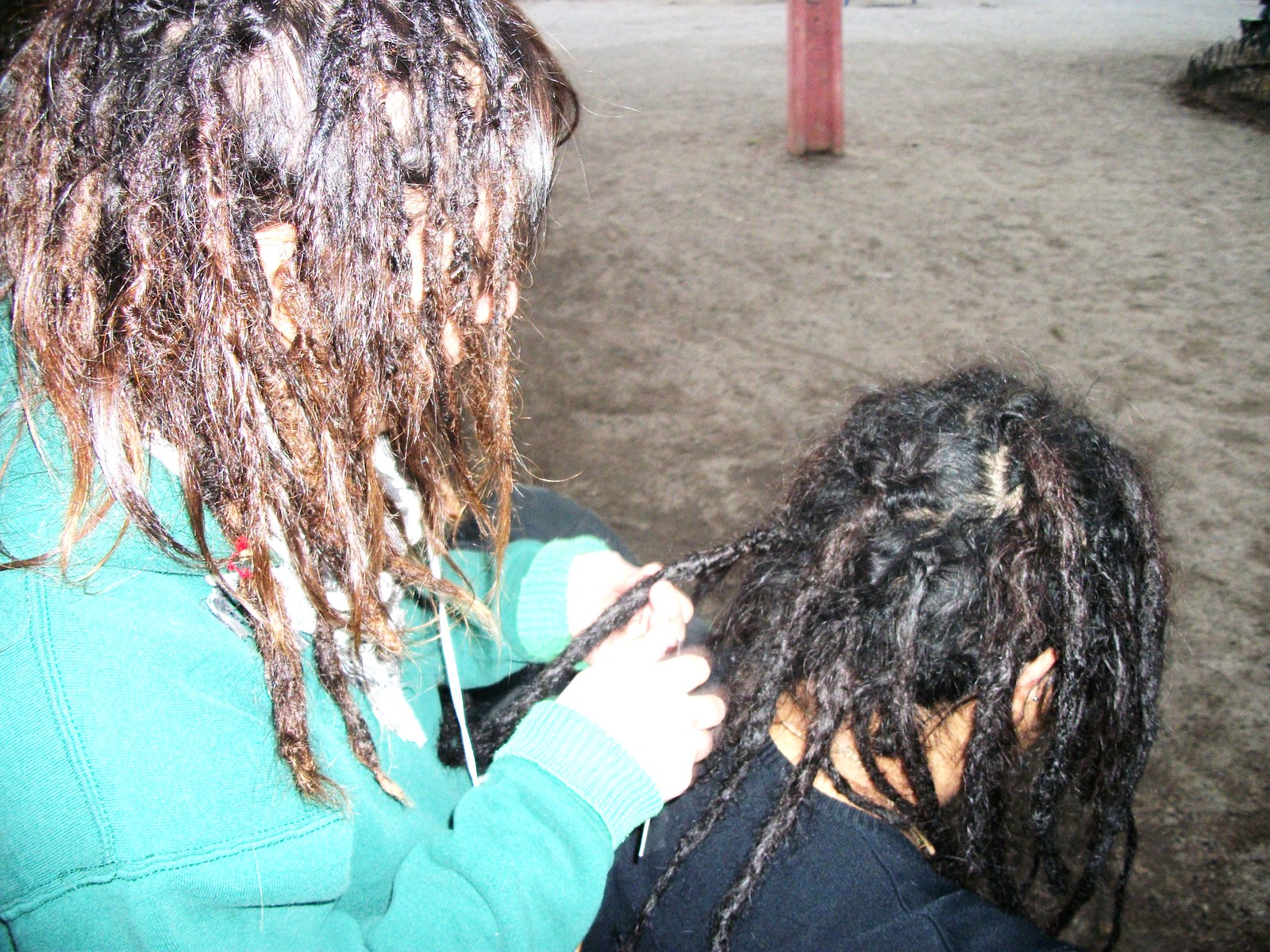This outdoor photograph, set against an earthy backdrop of sandy, gravelly dirt, prominently features a red post in the upper center, possibly serving as a marker or support. The scene captures two individuals centered in the foreground: the individual on the left is fair-skinned and wears a light teal sweatshirt. They have brown dreadlocks and are meticulously working on the dark dreadlocks of the person in front of them, who is seated and looking forward, partly obscured but wearing a blue sweatshirt. The overall setting suggests a casual, open space, possibly near a beach, with soft natural tones and textures contrasting with the vibrant colors of their attire.